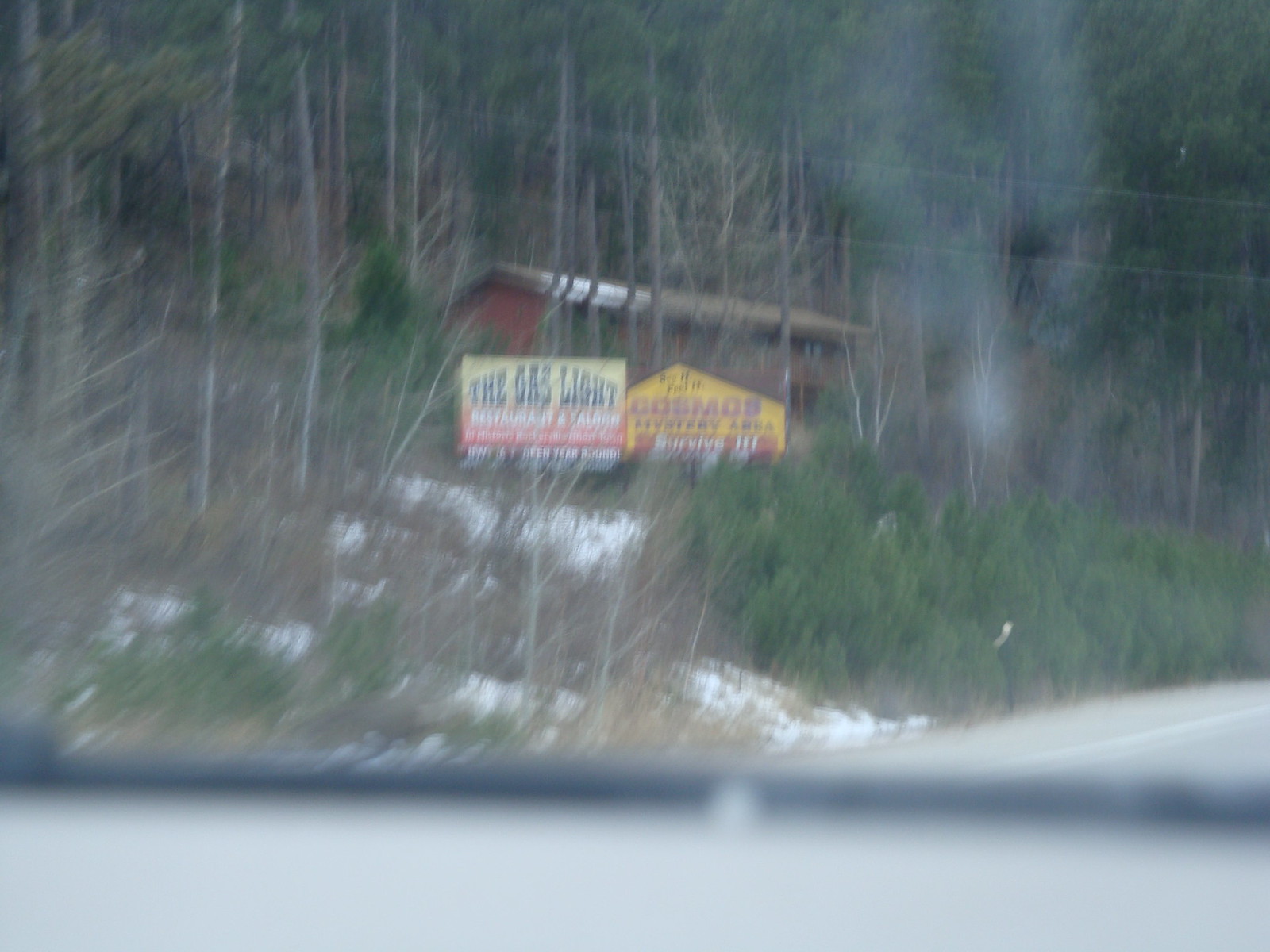This blurred photograph captures a reddish-brown wooden structure with a wide roof. The building has several windows and is surrounded by dense tree coverage, with some trees barren and others sporting green foliage. A power line runs across the scene. In the foreground, two billboards are visible. One of them, in black font, reads "The Gas Light" with additional white text below. The other billboard is yellow and displays the word "COSMOS" in a faded font, followed by some white text.